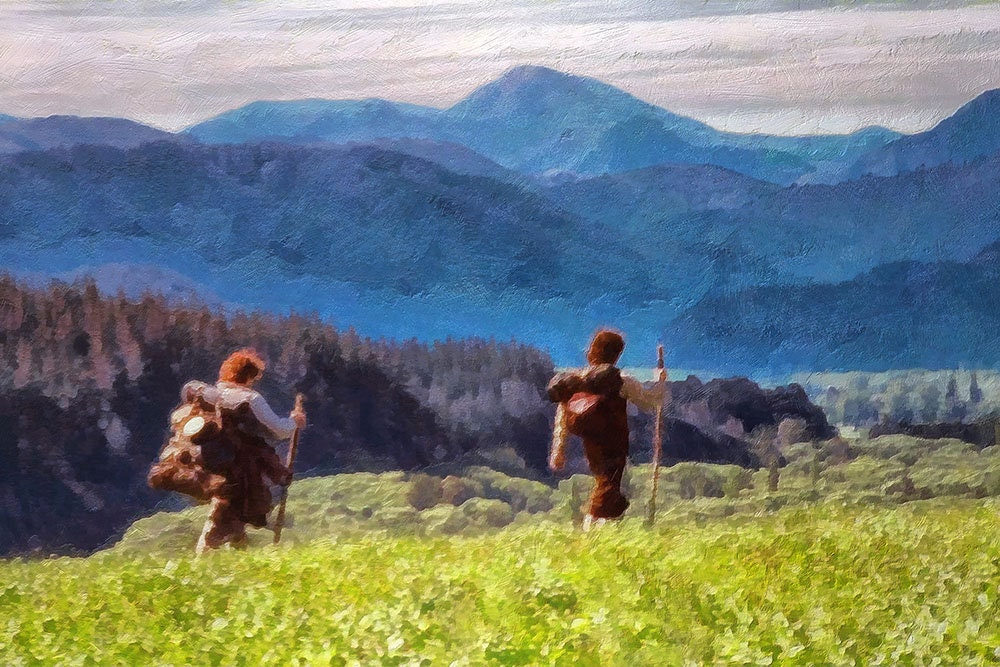This painting showcases two hikers journeying through a diverse landscape that extends from grassy fields in the foreground to towering mountains in the distance. The two figures, evocative of characters from "The Lord of the Rings," traverse a sunlit, rolly grassy field. They are encumbered with walking sticks in their right hands and backpacks, with the rear hiker bearing an especially large and overflowing pack. Both hikers sport brown hair and wear practical hiking attire; the hiker in front is clad in brown pants and a shirt, while the one behind wears dark pants and a white shirt, distinguished by his red fuzzy hair.

Surrounding the hikers is a picturesque and varied terrain. Immediately past the grassy expanse lies a rocky surface, leading into a densely forested valley adorned with rows of pine trees on hilly terrains. The trees at the edge of this forest are noticeably darker, indicating they are cast in shadow, while patches where the sunlight breaks through make the foliage glow brilliantly. The undulating land culminates in multiple mountain ranges, with the nearer ones appearing dark and hilly, transitioning to farther peaks dusted with snow and glowing lighter in the distance. Above all this stretches a dynamic sky, painted in shades of grey-pink with streaks of blue and purple hues mingled with clouds, creating a stunning atmospheric effect that envelops the entire scene.